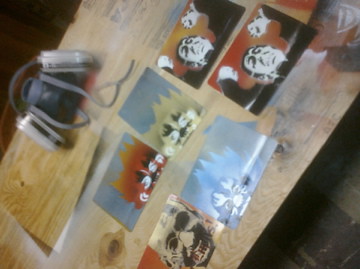This color photograph, although very small and low resolution, provides a fascinating glimpse into a wooden table adorned with various intriguing items. Oriented currently at a skewed angle, with its bottom left pointing down at an 8 o'clock position and the top right at a 2 o'clock position, viewers must tilt their heads to the left to correctly interpret the scene. The table, made of light-colored wood that resembles beech, shows distinctive knots and black-gray areas.

On this wooden surface, several objects are scattered. At what would be the top left corner in a corrected orientation, a pair of white headphones lies beside a black object, possibly a Walkman or tape player, with gray cords wrapped around it. The predominating colors on the table are red, black, white, blue, orange, and yellow.

Beneath the headphones are various photographs or postcards. One striking image depicts a frightening face with missing teeth or bloodstains, suggesting a menacing presence reminiscent of Dracula. Next to it, a wartime-like image from 1945 shows an angry man with raised fists, styled in a way that echoes Communist propaganda posters—his white flesh stark against a largely silhouetted form. Additionally, there are bright images potentially depicting celestial themes or portraits, including a smiling face that could be Gandhi's, plus a couple of ambiguous, possibly cat-related images.

The detailed assortment of these items against the wooden backdrop creates a vivid, albeit eerie, domestic tableau.